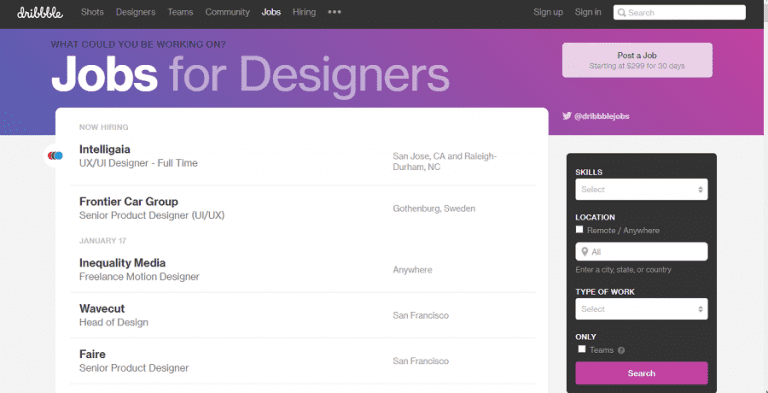The image depicts the job section of the Dribbble website, an online platform popular among designers. The webpage showcases several interactive elements and navigational options. On the top right, there are "Sign Up" and "Sign In" sections, accompanied by a search bar. To the left, the header features various categories, including "Shots," "Designers," "Teams," "Community," "Jobs," and "Hiring." 

In this particular view, the "Jobs" section is selected, highlighted by the title text: "What could you be working on? Jobs for designers." Directly beneath this, there's a prominent call-to-action button labeled "Post a job starting at $299 for 30 days." Additionally, a Twitter link for Dribbble Jobs is visible.

The main content area displays a list of job postings. The first five visible listings include:

1. **Intelligaya** - UX/UI Designer, full-time positions in San Diego, California, and Raleigh, Durham, North Carolina.
2. **Frontier Car Group** - Senior Product Designer, UI/UX, based in Gothenburg, Sweden.
3. **Any Quality Media** - Freelance Motion Designer, position available remotely.
4. **Wavecut** - Head of Design, located in San Francisco.
5. **Fair** - Senior Product Designer, based in San Francisco.

Additionally, the interface provides options to filter job listings by skills, location, remote work availability, city, state, country, and type of work.